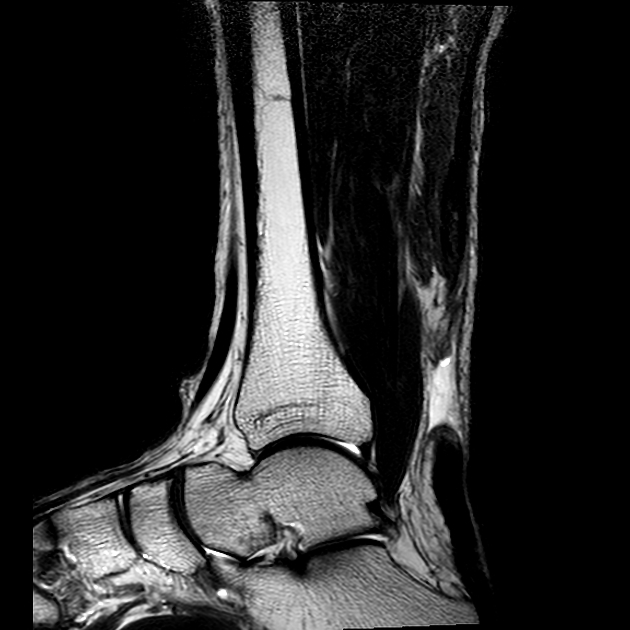This image depicts an x-ray of an adult human's ankle and foot. The image is characterized by a black background with the bones appearing prominently in white. At the bottom of the image, various bones of the foot are visible, ascending to the larger tibia bone in the lower leg, which is centrally positioned and extends upwards. On the right side of the x-ray, there is a faint outline that suggests the presence of skin and muscle. The alignment of the bones appears peculiar, indicating a possible injury, particularly around the heel or Achilles tendon area. This noticeable misalignment or disruption suggests damage, potentially to the Achilles tendon or another part of the ankle's structure. The focus and clarity on the bones suggest the image is an x-ray, despite some confusion due to the gray areas and overall monochromatic scheme.